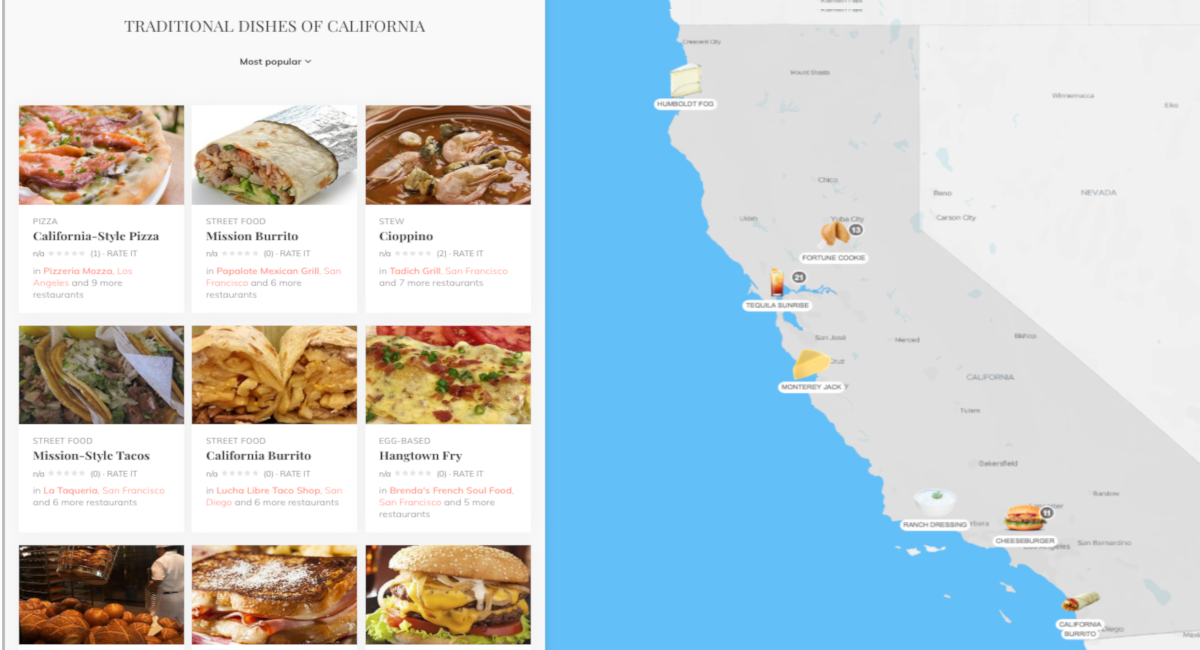The image appears to be a map featuring various food items, likely from California, depicted in a blurry manner. The map is divided into sections differentiated by two shades of gray, with water bodies also visible. The words "San Jose" or "San something" as well as "California" can be discerned, though not clearly.

Prominently featured in the image are traditional California dishes, including a California burrito and what appears to be a cheeseburger with identifiable ingredients such as a bun, green lettuce, and red ketchup, despite the overall blurriness. There's also a cup of ranch dressing with green herbs on top.

The left side of the image displays a legend or list describing various dishes:
- In the first row, first column, "pizza, California-style pizza" is mentioned.
- The next entry lists "street food, Michigan burrito."
- Following that is "stewed chopped peanuts, I-O-P-P-I-N-O."
- Another entry notes "street food, Michigan-style tacos."
- There's another listing for "street food, burrito, California burrito."
- Lastly, there is a reference to "egg base" or possibly "meat base," followed by "hangtown fry."

Overall, the image is a gastronomic exploration of California, albeit in blurred visuals, depicting popular and traditional dishes with a particular emphasis on regional street foods.